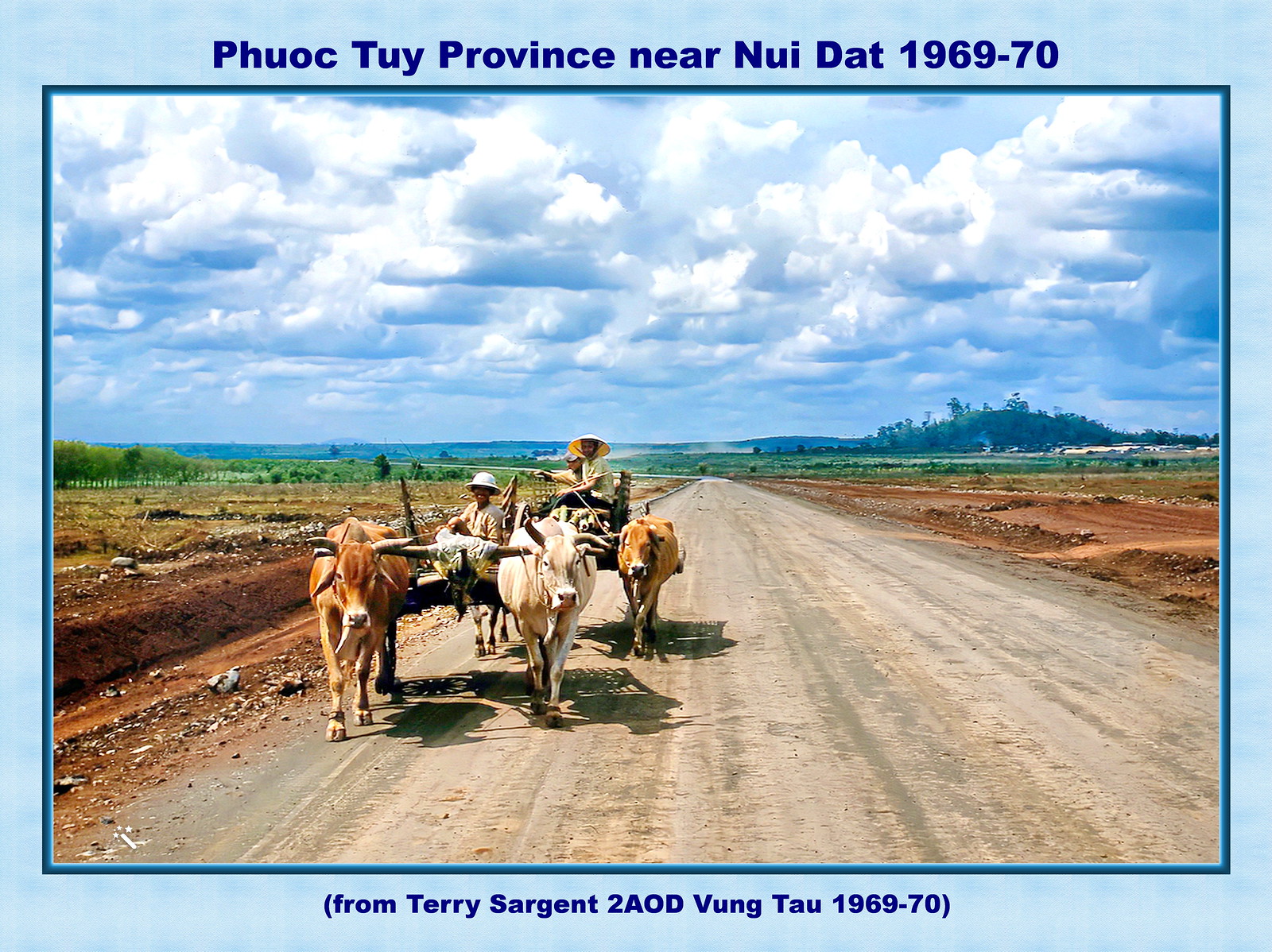The image depicts a detailed countryside scene, evoking elements of nostalgia and tranquility typical of traditional rural landscapes. At its center, a well-maintained dirt road stretches into the distance, bordered by wide, open fields and patches of grass. This road is traversed by a makeshift carriage drawn by three bulls, with a fourth cow walking alongside. The carriage carries three men, who are dressed in traditional attire and sporting large, rice paddy hats, indicative of Southeast Asian cultures. In the background, a sprawling landscape of fields meets the horizon where a distant ocean can be discerned, framed by formidable mountains under a vast, blue sky dotted with numerous white clouds. The image is identified by text at the top, reading "Phuoc Toi Province near Nui Dat 1969-1970 from Terry Sergeant 2AOD Vung Tau 1969-1970", giving it a historical context, possibly of an old painting or photograph from the Vietnam War era.